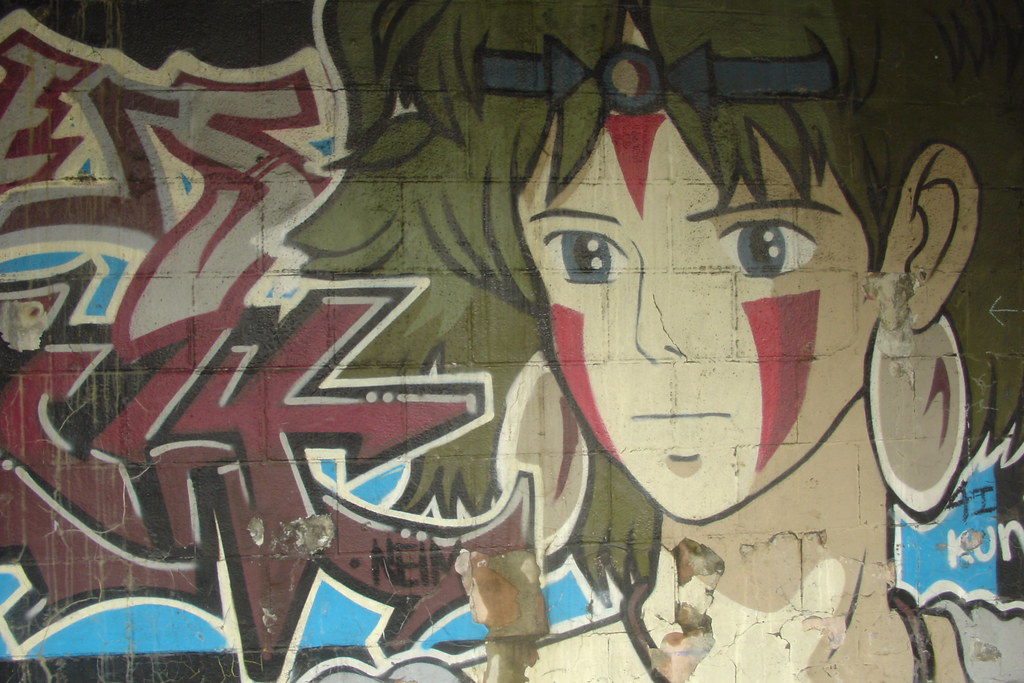The image features a horizontally aligned rectangular close-up of a stone wall adorned with vibrant graffiti. Dominating the right side of the picture is an anime-style cartoon character reminiscent of Japanese animation. The character sports long, spiky green hair outlined in black, a black headband, and a large earring. Their face is decorated with striking red triangular markings: one inverted triangle between the large blue eyes and two more on each cheek. The character's expression is neutral, with a straight line for a mouth and a small curved line suggesting a dimple on the chin. The figure is dressed in a gray shirt and looks towards the left side of the image, where bold, curvy graffiti lettering in gray and red fills the space. Among the letters, the artist's signature "M-E-I-M" is noticeable, along with another marking "4-I-K-U-N" in the lower right corner of the mural.